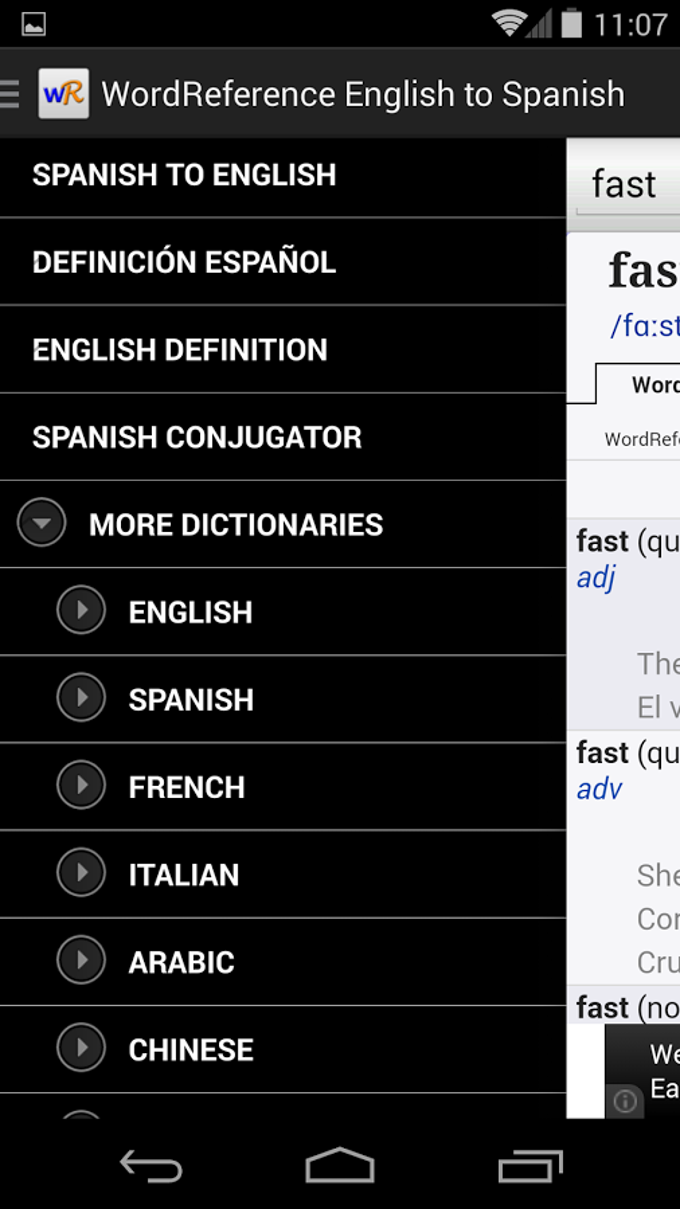Screenshot of a phone displaying an older user interface. At the top of the screen, there is a black banner featuring a picture icon in the left corner. Positioned to the right and almost centrally aligned are several icons: a fully connected WiFi signal, an empty signal strength icon, a fully charged battery, and the time reading 11:07.

Beneath this black banner is a slightly lighter one, which houses a faint, partially cut-off hamburger menu icon (three horizontal lines) on the left. Next to this, there is a noticeable white square with the initials "WR" inside—a lowercase 'w' in blue, followed by a gold uppercase 'R.'

The main content reads "WordReference" with subheadings "English to Spanish" and "Spanish to English," followed by "Definición Español" for Spanish definitions and "English definition." Further down, the interface mentions "Spanish conjugator" along with "More dictionaries," indicated by a dropdown arrow. The listed languages include English, Spanish, French, Italian, Arabic, and Chinese, each with an arrow pointing to the right.

On the far right side of the screen, there is partially cut-off text reading "Fast" along with other obscured information.